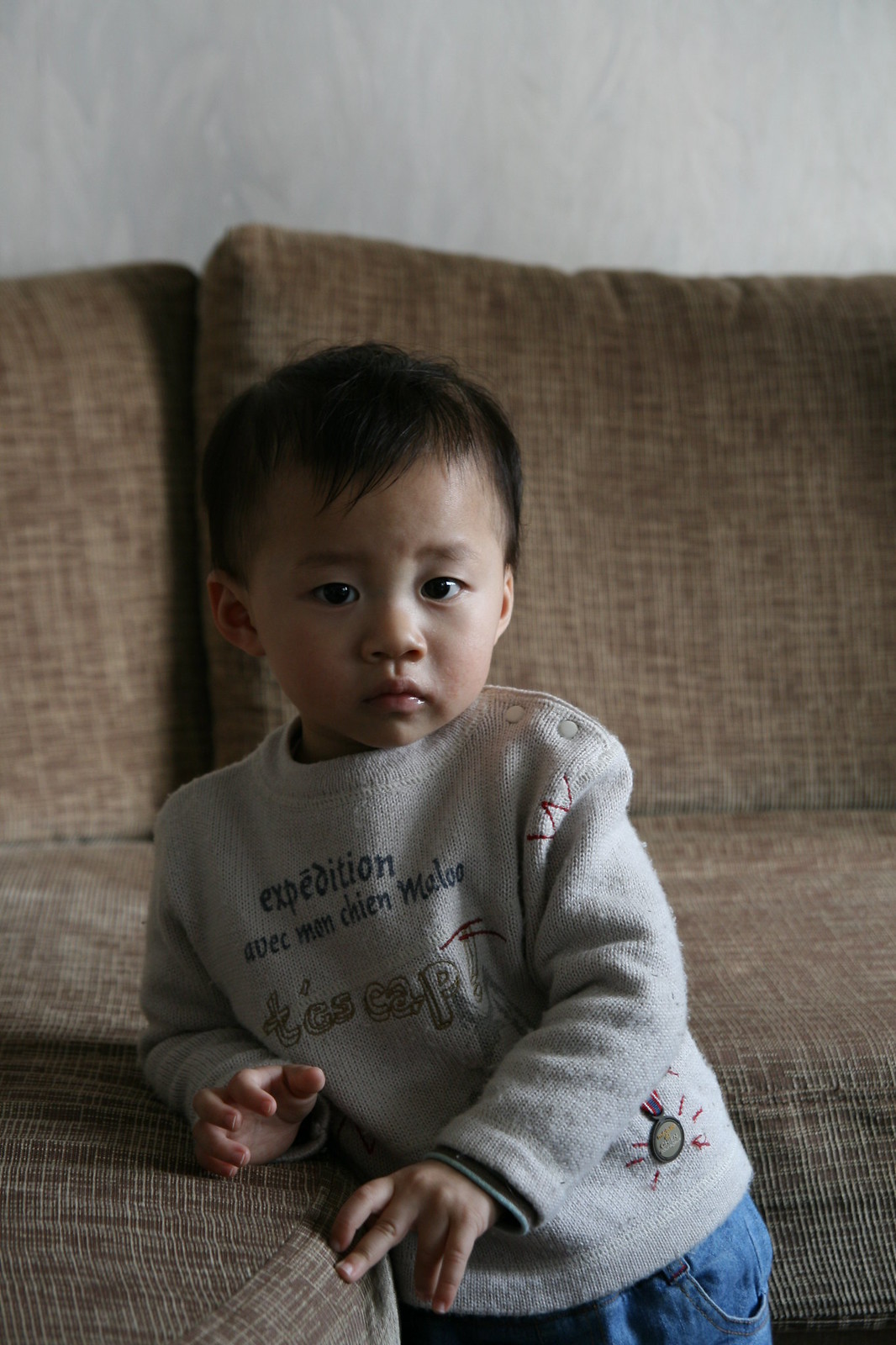The image portrays a young East Asian boy, possibly around 2 to 3 years old, standing in a living room with a textured white wall and sandwiched between two light brown fabric couches. The boy has medium-length, dark black hair that appears freshly cut. His face, illuminated primarily from the side, reveals a light brown complexion with an expression of concern or sadness as he looks directly at the camera. 

He is dressed in a grey t-shirt, which features the word "Expedition" in English, possibly containing additional symbols or text, and paired with light blue jeans. The boy’s posture involves his left arm resting on the brown couch, with two fingers of his left hand placed on top of a cushion and the other two hanging down. His right elbow props his forearm on the couch, his hand open and fingers slightly extended. The right side of his face is partially shadowed, making the details less discernible. The image is clear, high-definition, and sized approximately 8 by 10 inches.